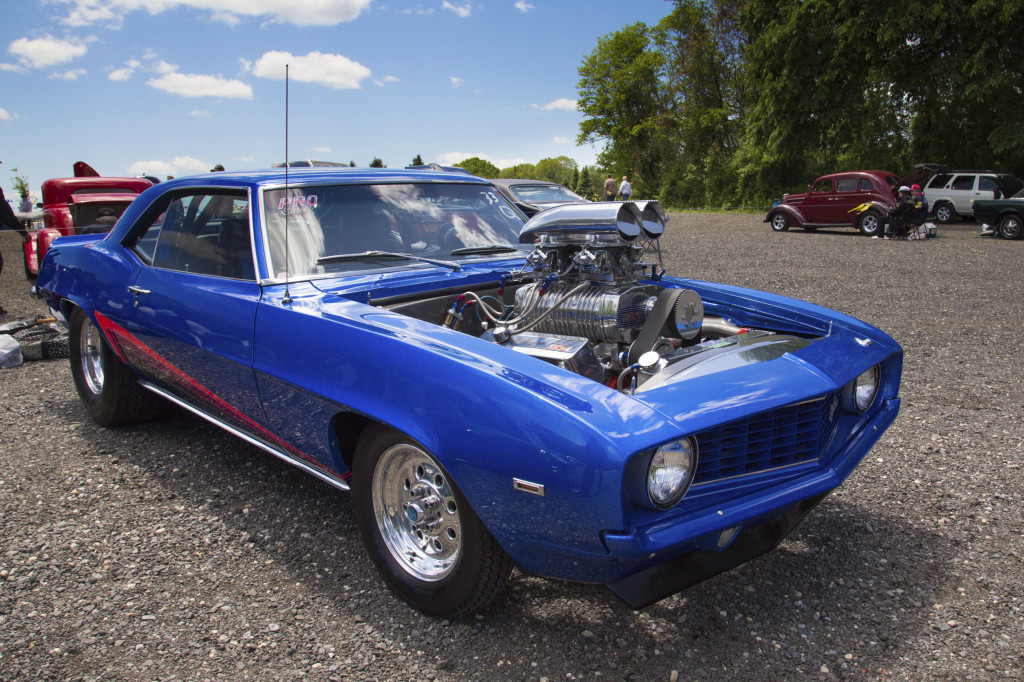This photograph captures a vibrant and dynamic scene at a classic car show. Dominating the center is a stunning royal blue sedan from the 1960s or 70s, with an eye-catching red stripe angling upward from the lower front side panel. The car's gleaming engine, protruding impressively from the removed hood, showcases its powerful build. It rests in a gravel parking lot, surrounded by other vintage vehicles, including a notable red 1927 Ford Coupe and what appears to be a maroon Volkswagen. The background is defined by a lush tree line under a partly cloudy daytime sky, adding a serene backdrop to the bustling display of automotive history. Two men can be spotted near the red Volkswagen, embodying the laid-back yet enthusiastic atmosphere of the car show.